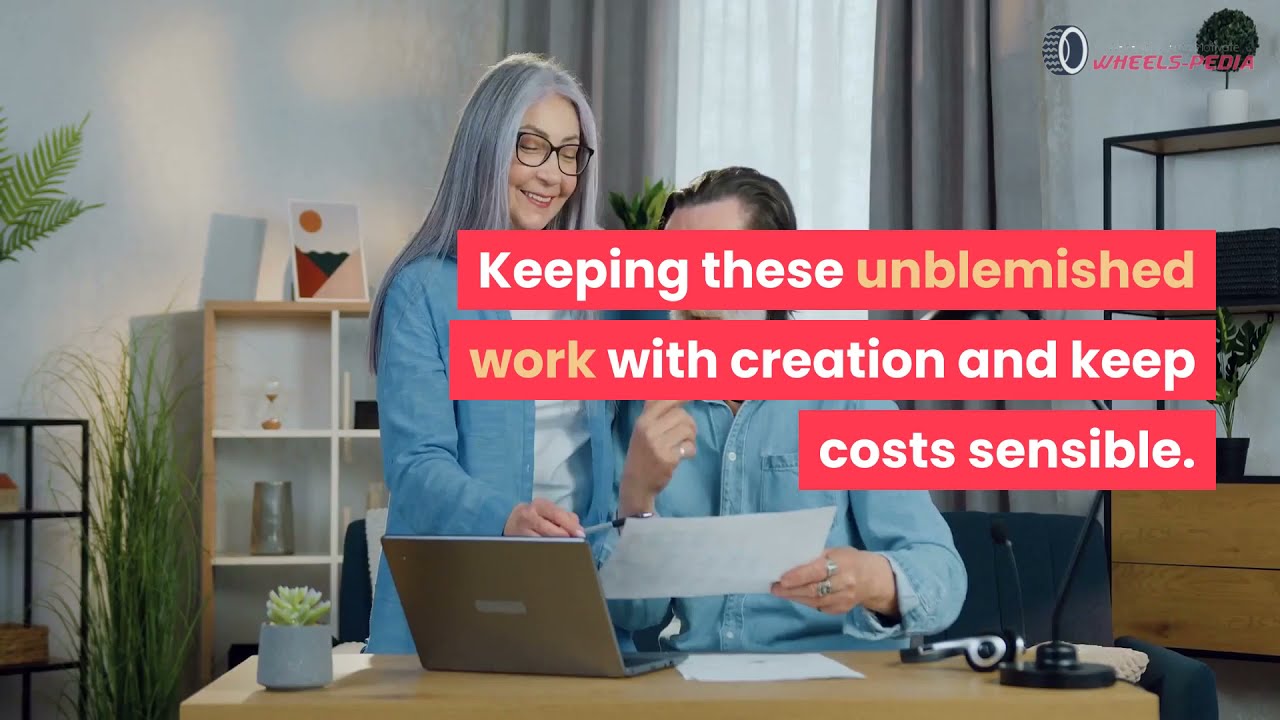In a cozy, well-decorated home office, a couple is immersed in their financial tasks. The couple, both wearing blue denim shirts, are focused on a piece of paperwork. The woman standing on the left, with long, silver-gray hair and black-frame glasses, points at the paper with a pen, smiling, while the man seated next to her holds the paper up. A banner with a red background and white and gold text obscures the man's face, bearing the message: "Keeping these unblemished work with creation and keep cost sensible." To the right top corner of the image, "Wheelspedia" is prominently displayed in pink lettering alongside a small tire icon. The room has a modern, laid-back vibe, with gray and white curtains, multiple plants, and shelving filled with an assortment of items. The couple appears content and satisfied as they manage their finances efficiently, likely with the assistance of Wheelspedia, as indicated by their organized workspace and cheerful demeanor.